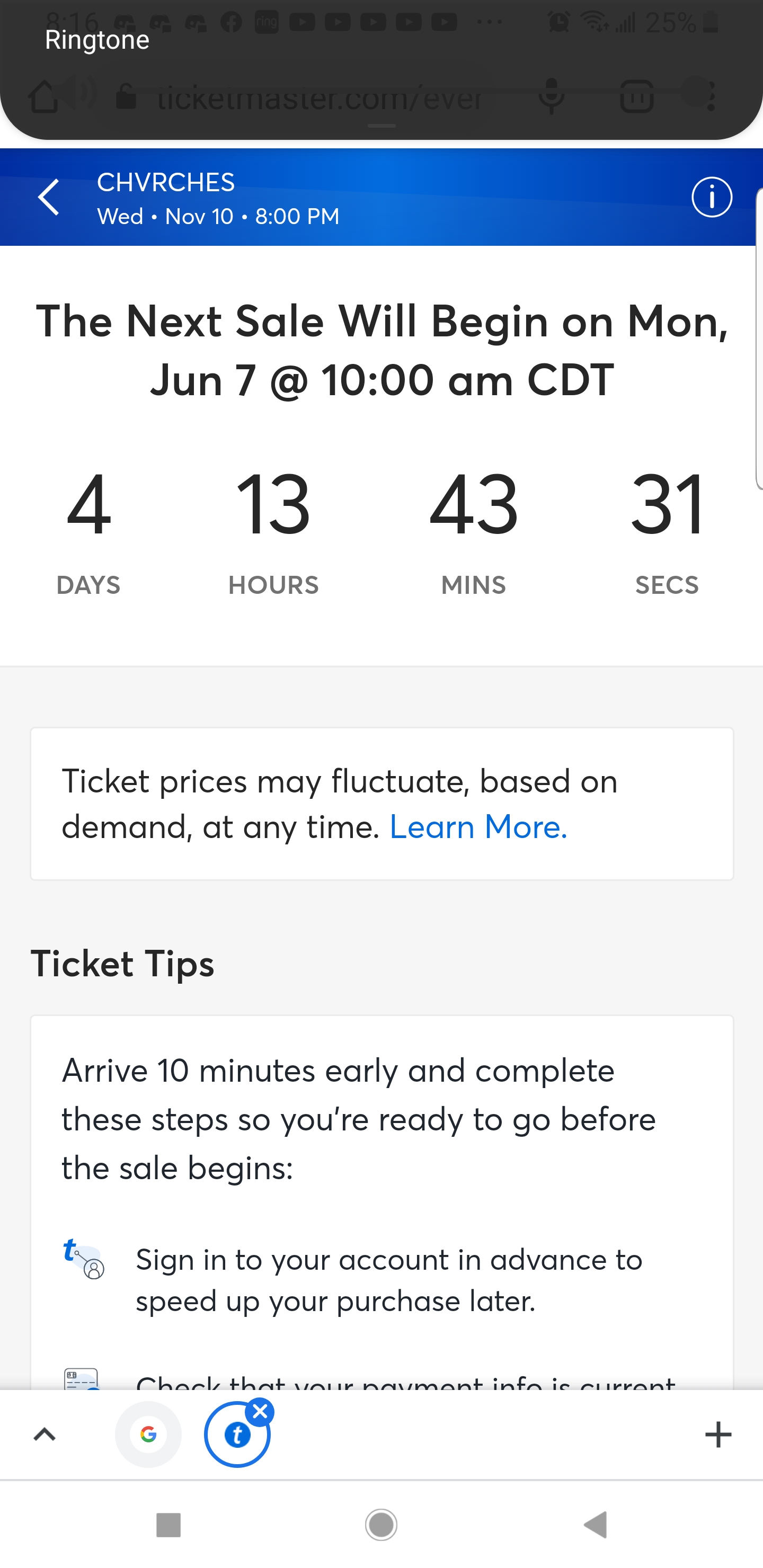The screenshot displays a website interface with several sections and details related to an event. At the top, a black bar with white text reads "Ringtone." Below this, there's a blue banner with a left-pointing arrow and white text announcing "CHVRCHES Wednesday, November 10th at 8 PM." On the far right of this banner is a white eye icon inside a white circle, presumably indicating more information.

Along the right edge of the screenshot, a vertical slider bar is visible. Beneath the blue section, black text informs that the next sale will begin on "Monday, June 7th at 10 AM CDT, Central Daylight Time,” along with a countdown showing "4 days, 13 hours, 43 minutes, and 31 seconds."

Further down, a gray box contains multiple white boxes. The first white box includes black text stating, "Ticket prices may fluctuate based on demand at any time," with a clickable "Learn more" link in blue. Below this, another segment titled "Ticket Tips" in bold black text is present.

The subsequent white box advises, "Arrive 10 minutes early and complete these steps so you're ready to go before the sale begins," with a corresponding symbol on the right side. Further tips include "Sign into your account in advance to speed up your purchase later" and "Check that your payment info is correct," each accompanied by relevant symbols. Additional icons such as a Facebook logo with an "X," a Google sign, and others are situated towards the bottom of the screenshot.